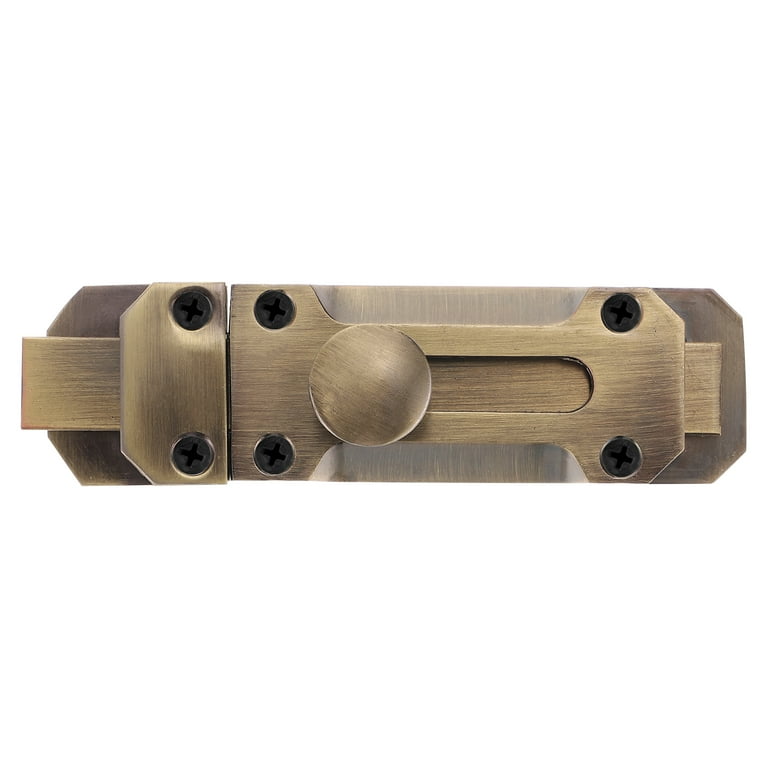The image showcases a detailed, metallic slider lock made entirely of brass, positioned against a pure white background. The lock comprises two main components: a short brass piece on the left and a longer brass piece on the right. The centerpiece features a round brass knob attached to a brass bar that slides within an elongated base to secure or release the lock. The longer right piece contains the knob and a mechanism allowing the bar to move back and forth. Black circular indentations are evenly spaced along the lock, each featuring a black screw, securing the lock in place. The entire piece has a brushed, grainy texture, giving it a shiny and reflective appearance. The lock, reminiscent of those used in hotel rooms, gives off an animated vibe, suggesting it may not be an actual lock but rather an illustrative or architectural depiction, possibly seen in a movie or catalog.